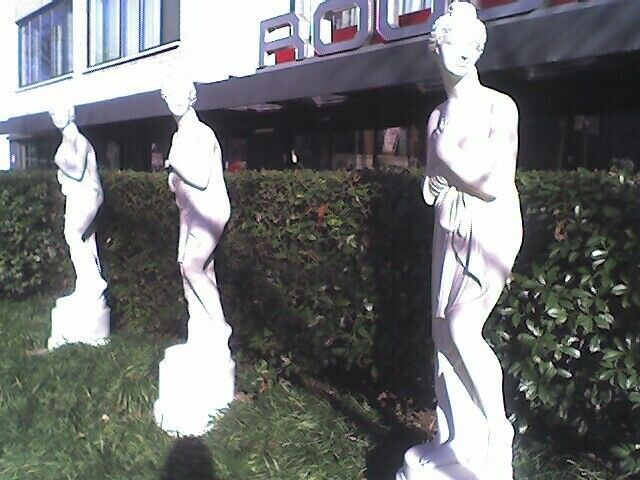The photograph captures a serene outdoor scene in front of a commercial building. In the foreground, three identical white statues of women are arranged in a line on a green lawn. Each statue features a woman with her hair in a bun, wearing a short-robed outfit, and holding a flowing piece of fabric over her chest. Their bodies are slightly slouched with shoulders leaning left, while their heads are bent towards the right. Behind these statues is a well-kept, dark green leafy hedge. Beyond the hedge, there is a building facade with large second-floor windows visible on the top left. Part of the building's name is discernible, featuring the letters "R-O-U" on the roofline, although the complete name and type of establishment remain unclear. The scene lacks the presence of people, animals, or mechanical objects, focusing purely on the tranquility and elegance of the statues and their surroundings.